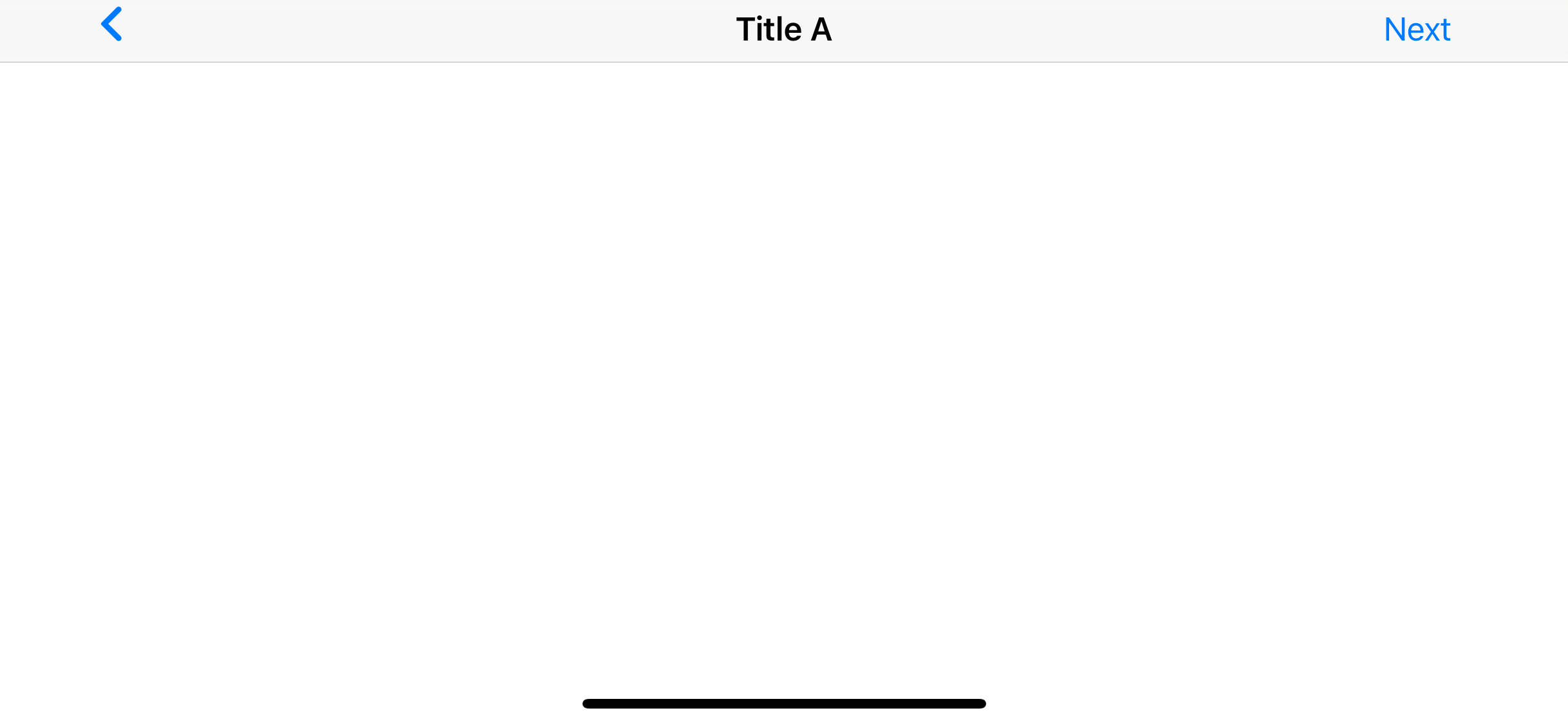The image is a simple, minimalist interface design, likely displaying a webpage or application screen in landscape orientation. The background is entirely white, blending seamlessly with the viewer’s white computer screen, making it challenging to distinguish the image’s boundaries. 

At the top, a pale gray horizontal bar stretches across the full width of the image. On the left side of this bar, a blue, left-facing arrow is visible, suggesting a "back" or "previous page" function. In the center of the gray bar, the text "Title A" is displayed in a black, sans-serif font resembling Arial. The word "Title" begins with a capital T, and "A" is also capitalized. On the far right of the bar, the word "Next" appears in the same blue color as the arrow, but it is in a regular weight, contrasted with the boldness of the title.

The rest of the image is stark white, devoid of any other elements or text, except for a single thick, bold black horizontal line. This line is centered in the image, occupying the middle third, though exact margins are indiscernible due to the uniform white background. The overall design emphasizes minimalism and clarity, focusing on navigational elements without any additional content or distractions.